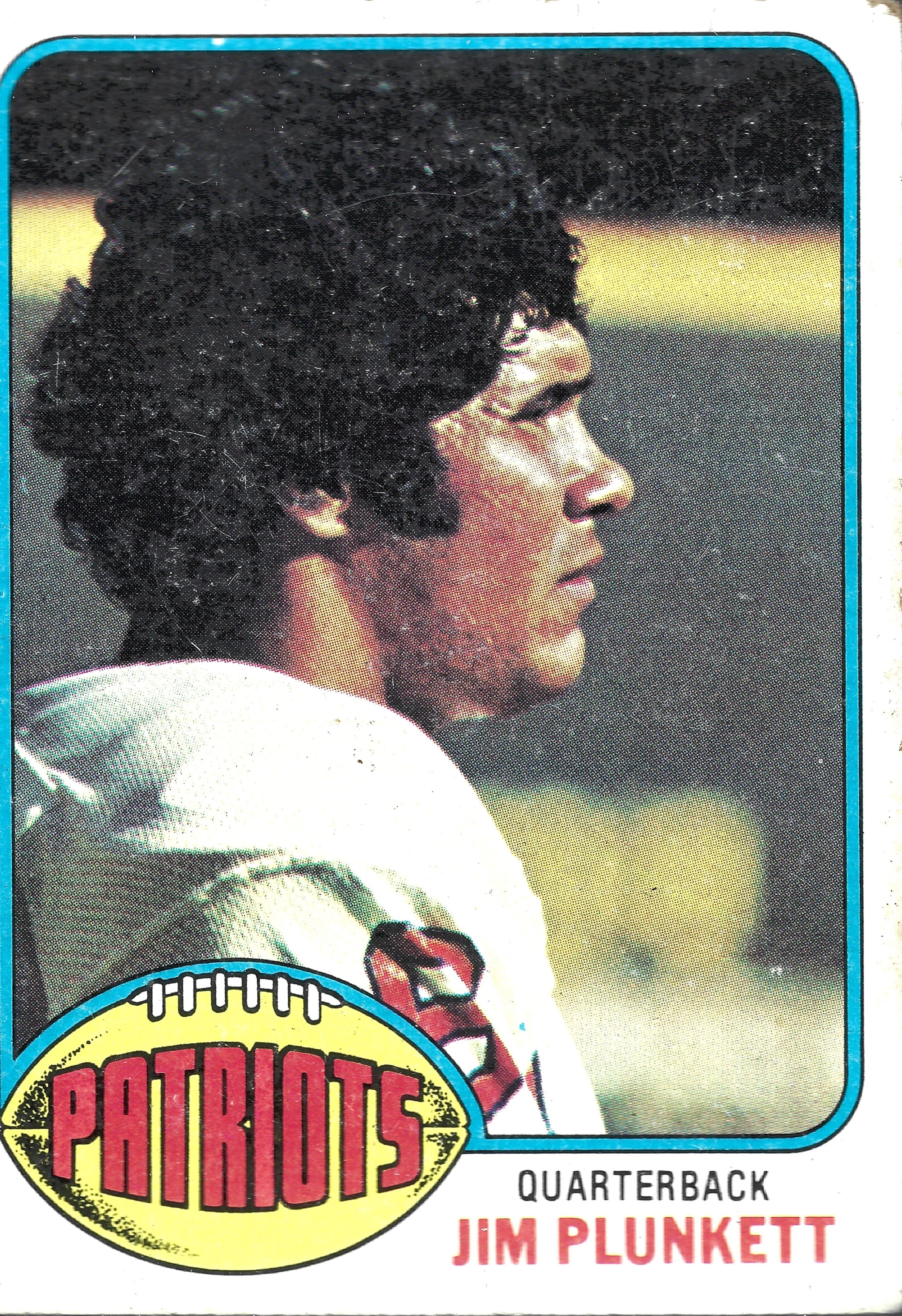This is a vintage football trading card set outdoors, showcasing a profile photograph of Jim Plunkett, a white man with abundant black hair and sideburns extending to his ear. Clad in a white jersey adorned with the red number "six" or "nine," he stands against a backdrop featuring a gray wall accented with a yellow stripe. Prominently displayed at the top of the card is the word "Patriots" inside a yellow football icon. Further down, the text in red spells out "Jim Plunkett," while "quarterback" appears in black. Judging by the design and details, the card seems to originate from the 1970s.